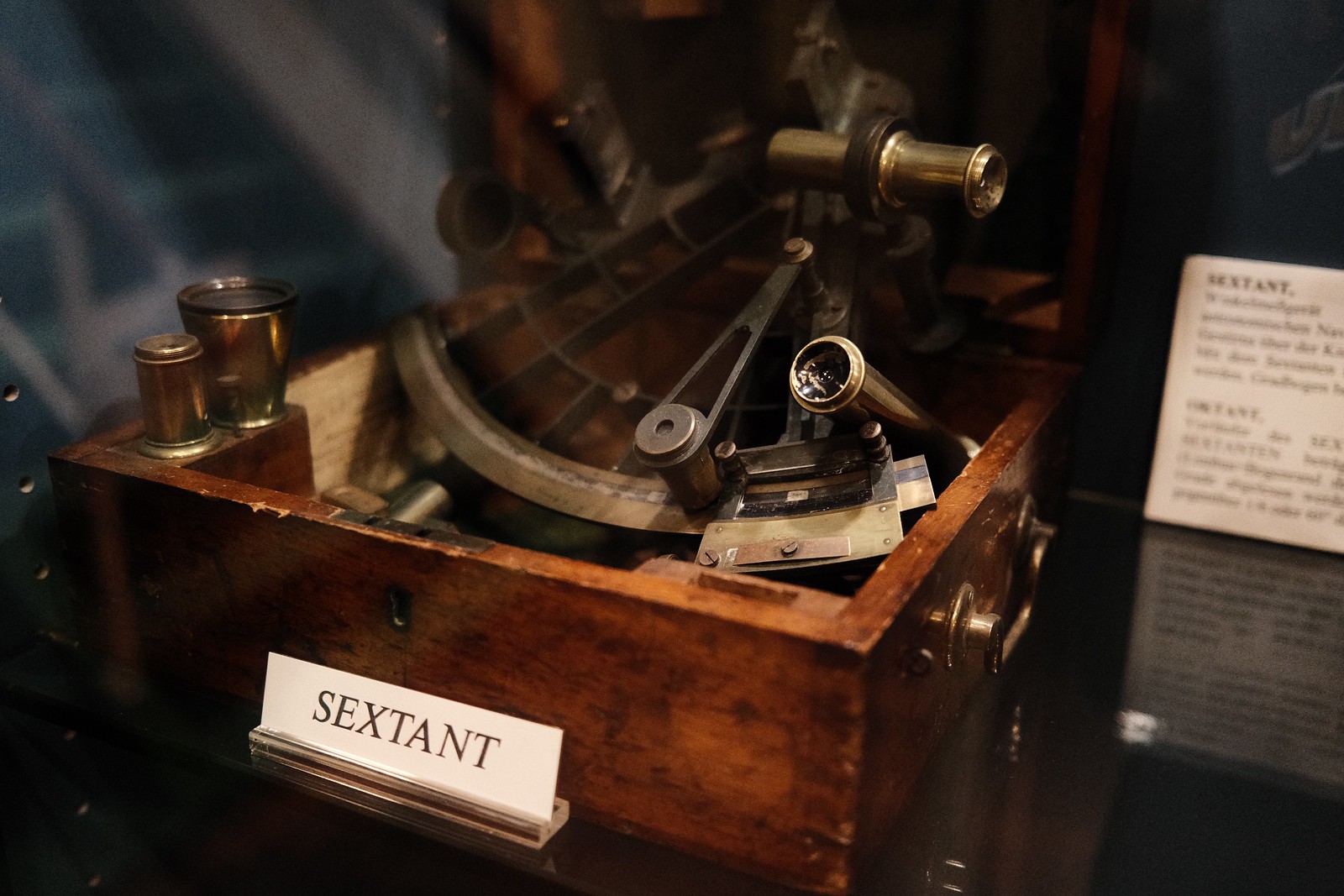The image depicts an indoor setting, likely within a museum, showcasing an old sextant housed in a worn, square wooden box with an antique finish. The wooden box, possibly a repurposed drawer due to the golden handle visible on its right side, sits atop a reflective, shiny surface, perhaps a glass table. The sextant itself, composed of brass and gold-colored metal components, features intricate details such as an eyepiece and several small cylinders. Directly in front of the sextant, a white placard bearing the word "Sextant" in black font is displayed on a clear stand. To the right of the box, an additional white card provides further information about the sextant, though its text is blurry and unreadable. The background hints at a museum setting, possibly indicated by what appears to be a staircase, cementing the notion that this is a detailed exhibit designed to educate viewers on the historic navigational instrument.